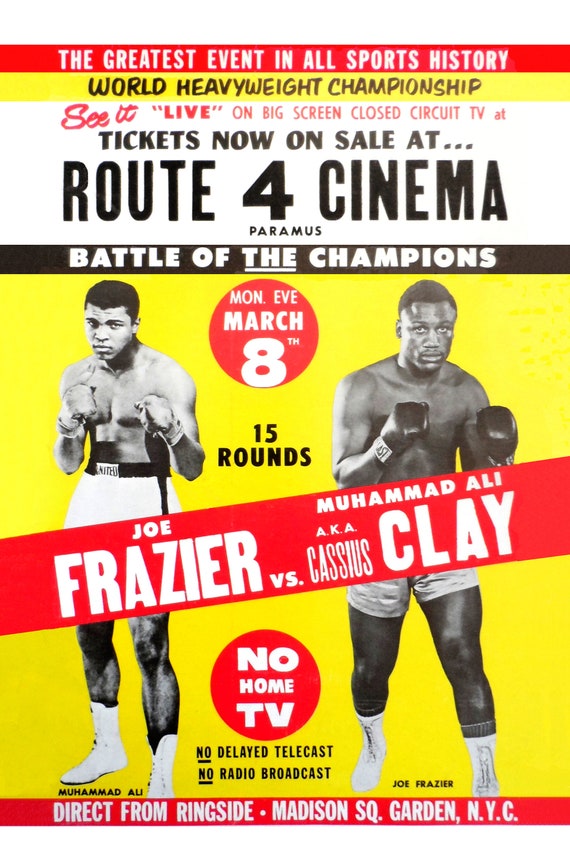This poster promotes an iconic boxing match between Joe Frazier and Muhammad Ali, also known as Cassius Clay. Dominated by bold yellow and red colors, the poster announces "The Greatest Event in All Sports History" and "World Heavyweight Championship." At the very top, a strip of white features these proclamations in red and black text. 

In the center, against a yellow backdrop, there are black-and-white photographs of the two boxers, each with fists up and poised for action. Interestingly, the images are swapped: Joe Frazier's name is placed above Muhammad Ali's photo and vice versa. A red ribbon with white text prominently reads "Joe Frazier vs Muhammad Ali aka Cassius Clay." Both fighters stare intently at the camera, wearing boxing trunks.

At the bottom, the poster has another white section with red and black text that reads "See It Live on Big Screen, Closed Circuit TV," and specifies that tickets are on sale at Route 4 Cinema, Paramus. Additional information includes "Battle of the Champions, Monday Evening, March 8th," and details about the 15-round match. It emphatically states “No Home TV, No Delayed Telecast, No Radio Broadcast," emphasizing the exclusivity of the live event, which will be broadcast "Direct from Ringside, Madison Square Garden, New York City."